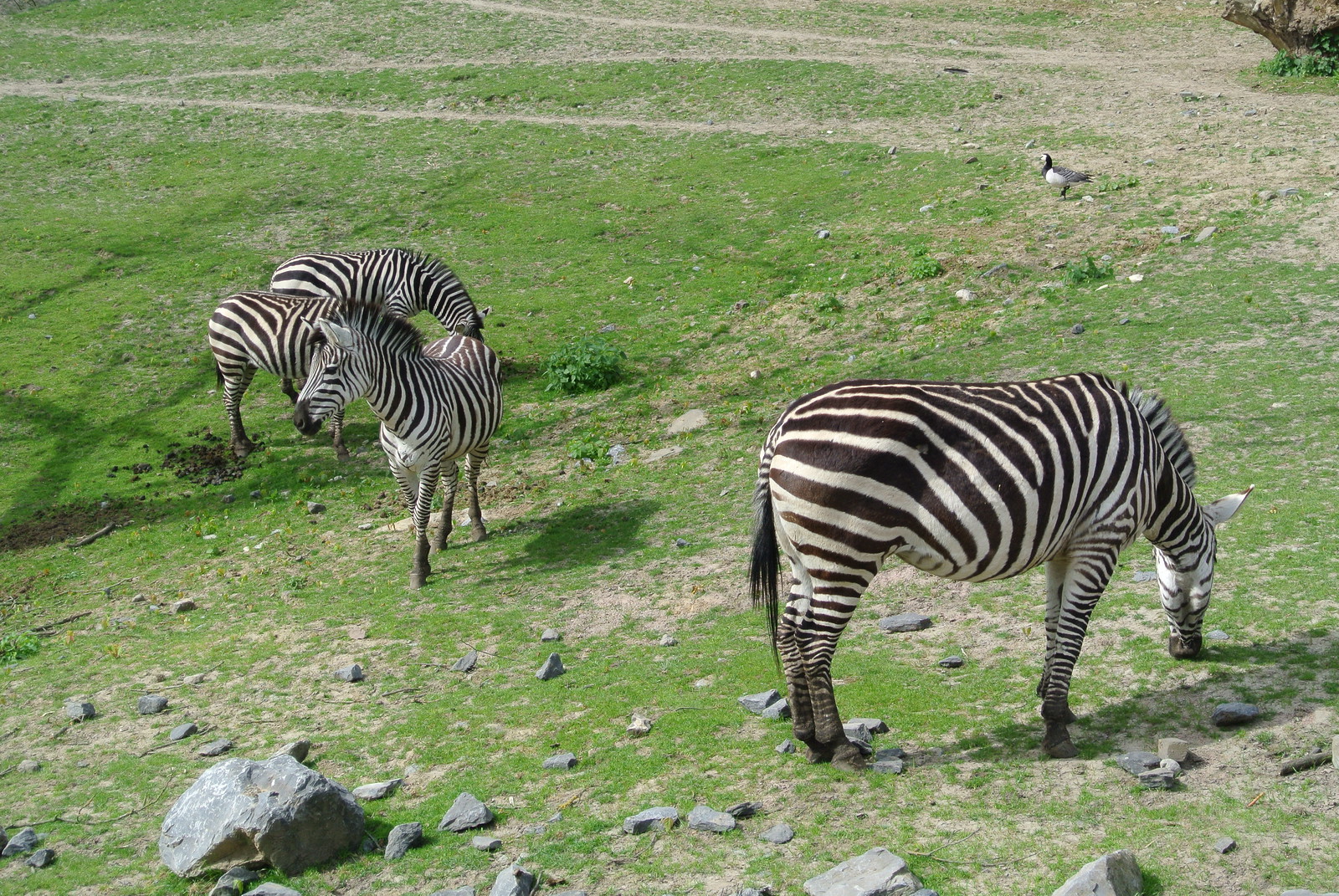In this outdoor photograph, the scene is set in a vast field of short green grass, interspersed with rocks and tiny bushes. Four zebras occupy the frame. On the right side, a large zebra stands alone, its head lowered as it grazes. To the left are three other zebras; the one in the front is walking leftward with its side profile visible, while the two behind it graze with their heads down, showing only their bodies and a bit of their necks. Additionally, a small bird, gray with a white belly, is perched near the edge of a gravel trail in the upper right corner. The background also features a tree limb and a dead tree stump, adding natural complexity to the serene landscape.